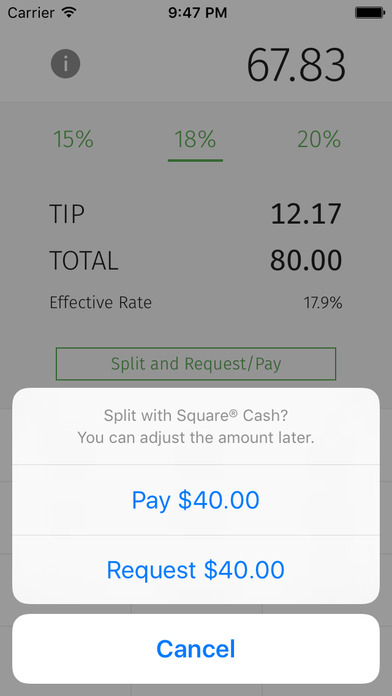Screenshot from a Mobile Bill Splitting App

The image is a detailed screenshot from a mobile app designed for bill splitting and payment management. The user interface is neatly organized, with the top bar displaying essential status information: the carrier is on the left, the current time, 9:47 p.m., is centered, and the battery status is on the right.

The main screen prominently shows the bill's total amount as $67.83. Below this, there are options for selecting tipping percentages, specifically 15%, 18%, and 20%. The 18% option is highlighted, showcasing a tip calculation of $12.17. Combining the bill total and tip, the overall amount comes to $80.00, reflecting an effective tipping rate of 17.9%.

Beneath the total amount, there is a prominently displayed button labeled "Split and Request Payment." Upon activation, a dialog box appears, providing options to split the bill with Square Cash. Users can adjust the split amount and have the flexibility to either "Pay $40" or "Request $40," with an additional option to cancel the process.

The interface is clean, straightforward, and user-friendly, offering essential functionalities for easily managing shared payments, whether dining out or engaging in various social activities.